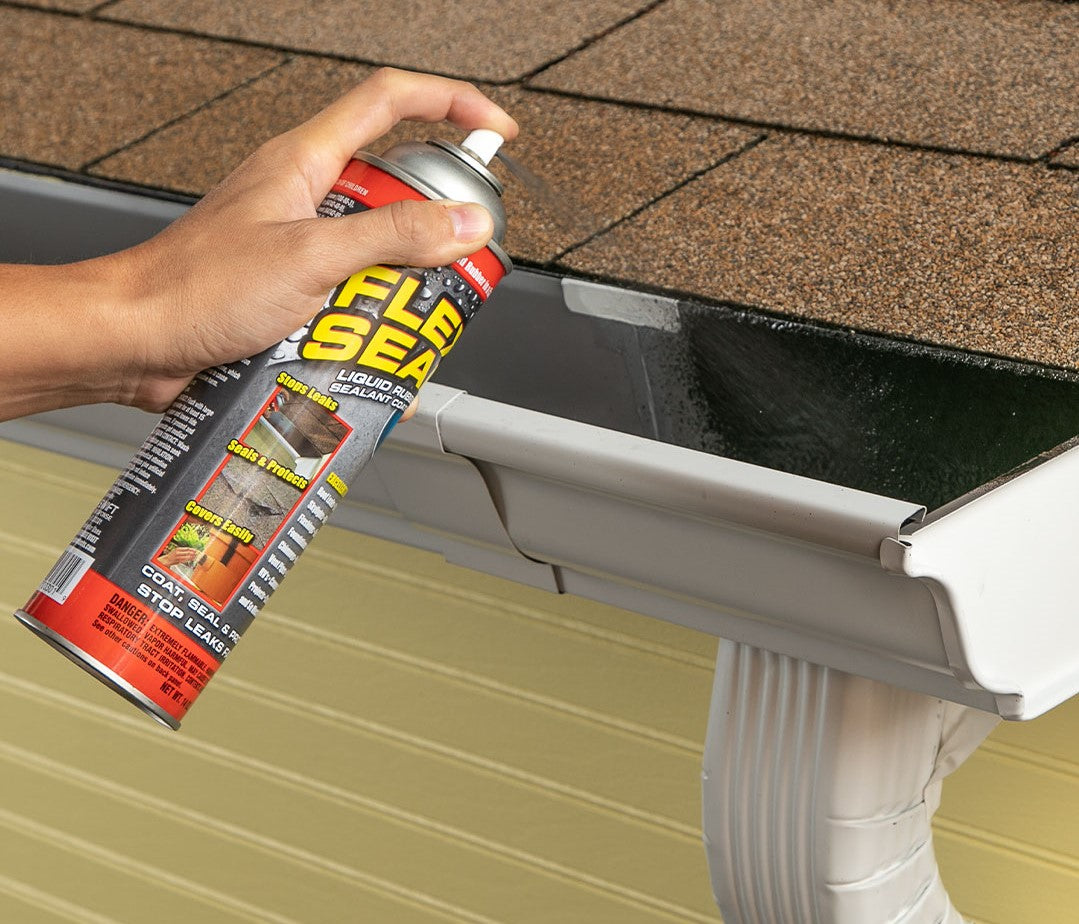The image is a detailed and colorful advertisement for Flex Seal, a sealant in an aerosol can. At the center of the square-format photograph is a white gutter attached to the edge of a house roof. The roof is covered in brown shingles, and the house has a light yellow lateral siding pattern. The gutter itself is white on the outside and dark gray on the inside. 

A left hand extends from the upper left corner of the image, holding and spraying the Flex Seal can into the gutter. The Flex Seal can, which prominently displays its name in bold yellow letters at the top, is releasing a black spray. This spray immediately turns the inside of the gutter from gray to black. The can also lists its uses down the side, including "stops leaks," "seals and protects," and "covers easily." 

In the bottom right corner, there is a white downspout connected to the gutter. The product's efficacy is being visually demonstrated as the black sealant covers and presumably repairs the area being sprayed. The image captures the action of the black spray clearly coming out of the nozzle and separating the newly blackened section of the gutter from the original gray interior. The photograph showcases the product's application in a realistic and representational style.